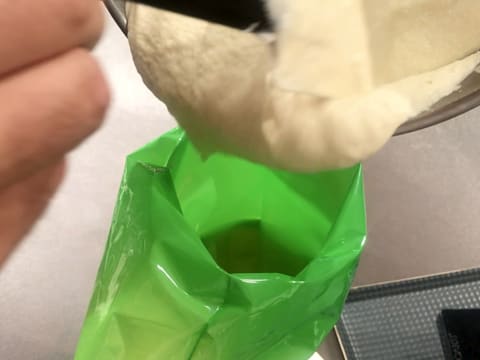In a laboratory setting, a person is carefully pouring a white cream or paste from a glass container into a very small green bag. The opening of the bag, held to the left by their fingers, appears to be about two fingers wide. The glass container, which is cushioned and stabilized with paper to prevent it from moving or breaking, is being tilted to transfer the substance. On the lower right-hand corner of the image, there is an unidentified device attached to some structure, whose purpose remains unclear. Additionally, there is a black tray located in the bottom right corner, possibly used for organizing and containing various scientific materials or samples. Overall, the action being depicted seems meticulous and precise, likely part of a scientific experiment or sample collection process.